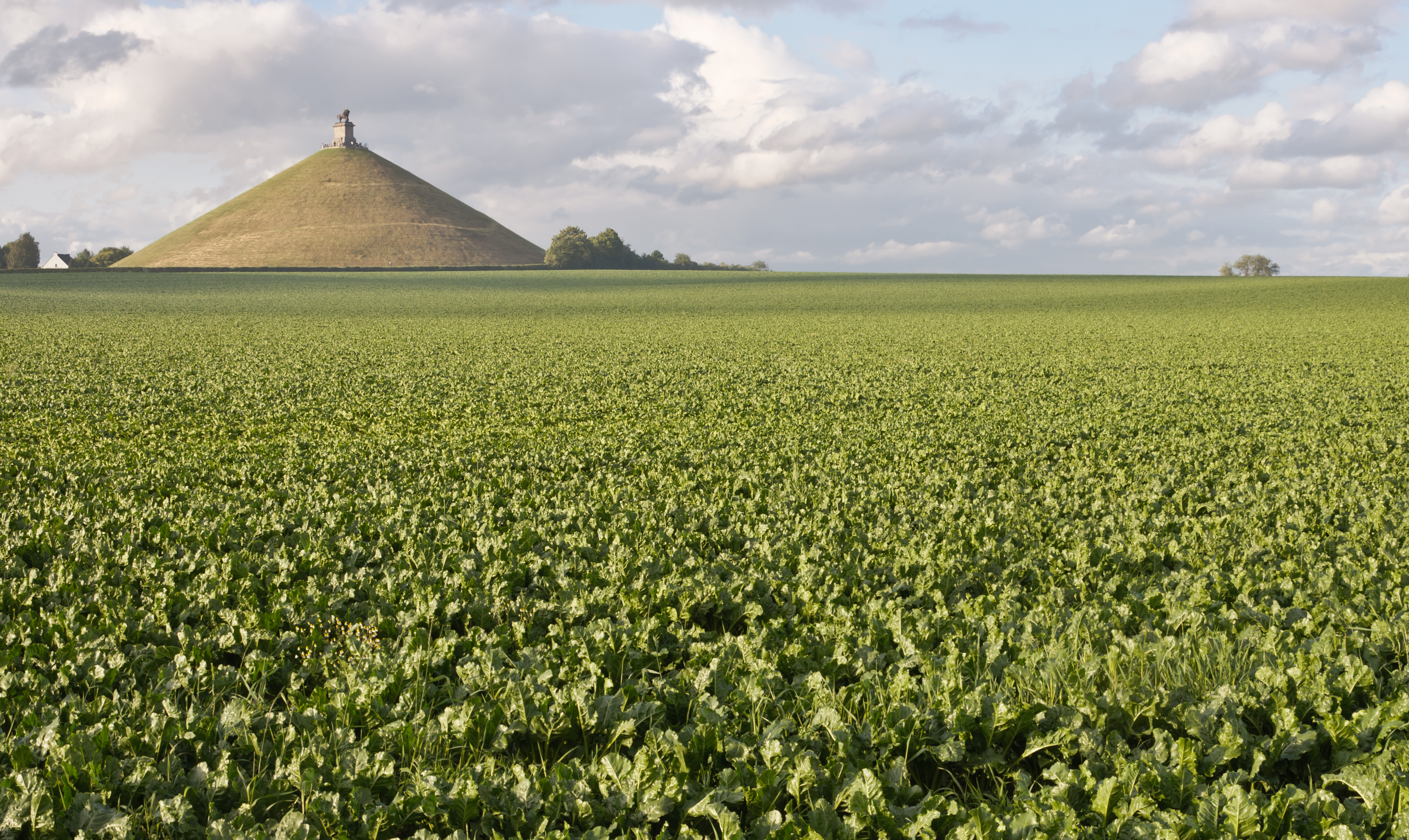This vividly colored photograph captures a sprawling field of lush green plants, likely a broad-leafed crop such as beets, with blades of grass interspersed in the foreground. Dominating the background is a prominent tan-colored mound, winding with a spiral path leading to a small gray building perched at its summit. The scene is set under a pale blue sky dotted with white and gray clouds, giving it an almost surreal quality. A smattering of trees lines the horizon, while the far-left edge reveals the dark roof and partial silhouette of a white house peeking from the distance, adding a touch of human presence to this picturesque landscape.